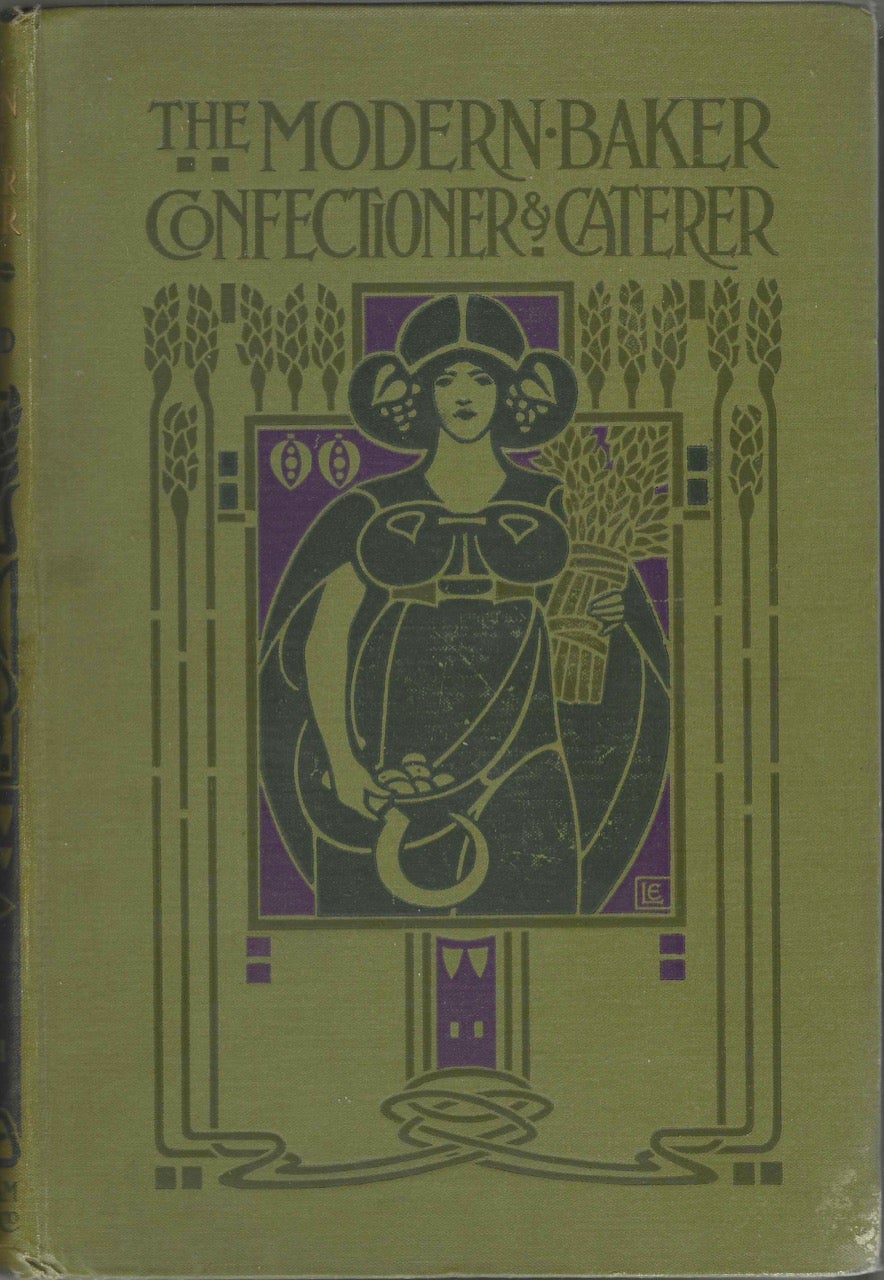This is a color photograph of the cover of an old cloth-bound book titled "The Modern Baker, Confectioner, and Caterer." The book cover is predominantly olive green with intricate Art Nouveau designs. In the center, there is a prominent image of a woman dressed in black, adorned with a cloak and an ambiguous headdress. She holds a bundle of grain in one hand and a sieve or sickle in the other. The woman is set against a blue-purple background that encloses much of her figure, except for her head which extends into another blue, rectangular box outlined in dark green. Surrounding her are elaborate, stylized decorations featuring interwoven lines and wheat motifs, enhancing the overall elegance of the cover.